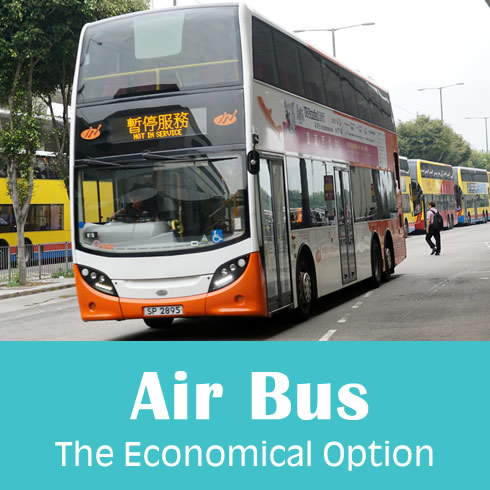This photograph captures a vivid urban scene featuring an Airbus double-decker bus prominently displayed on a city street. The sky is overcast with a white hue, and the background reveals lush green branches in the upper left, while the upper right shows additional trees and T-shaped streetlights.

At the heart of the image is the imposing front end of the Airbus, adorned with a large, clear driver's window, and a digital display in the middle. The display conveys a message in what appears to be Japanese or Chinese characters, alongside an English notation declaring "not in service." The bus itself is primarily white, accented with notable orange detailing, including an orange bumper. Its license plate, marked SP-2895, is clearly visible.

Flanking the main bus scene, a man with a black backpack and black pants is depicted crossing the street in the background, slightly blurred due to distance. On the opposite side of the street, several other buses, mostly in yellow with colorful red, blue, and black stripes and tinted windows, are orderly parked along the curb.

Completing the scene, a blue rectangular graphic beneath the bus emphasizes the promotional nature of the image. In large white letters, "Airbus" is printed, followed by the slogan "the economical option" in smaller, bold letters, all framed within the blue rectangle, underscoring the advertisement's message.